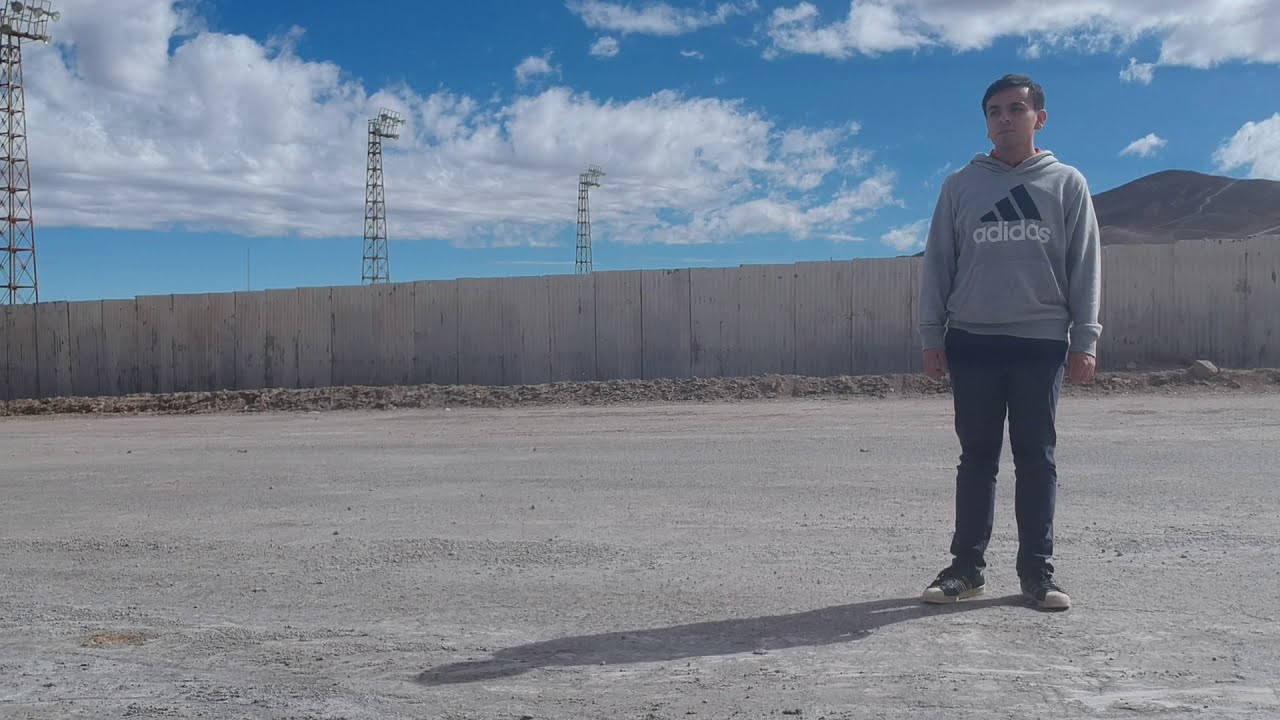A young man stands outdoors in what appears to be an unpaved road or city culvert, situated in a rural area. The ground beneath him is smooth and light grayish, with scattered rock piles. He is positioned slightly to the right side of the image, casting a long shadow in the late evening light. The man is dressed in a gray Adidas hoodie with a black and white logo, dark jeans, and black Converse-style sneakers with white tips. His arms rest casually by his sides, and he has short dark brown hair and lighter skin. 

Behind the man, a gray cement wall runs horizontally from the left to the right of the image. Beyond this wall, on the left side, there are various towers equipped with lighting fixtures, resembling those found in an industrial facility. Further in the background, a network of power lines stretches from the center-left towards the top left corner of the image. To the right, a tall hill or mountain rises against a backdrop of a partly cloudy evening sky. The overall scene is characterized by its calm and somewhat industrial yet rural atmosphere.